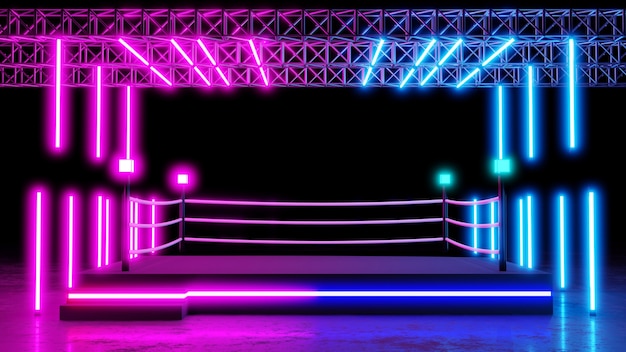The photograph captures a stage-like platform reminiscent of a boxing ring, framed by a captivating array of neon lights. The elevated platform, accessible by a single step, is bordered on three sides by ropes—like a boxing ring—but with an open front, inviting one to step up. Above, the scene is dominated by steel girders from which neon rods hang. The left-hand side glows with vertical pink neon lights, while the right is bathed in blue, creating a striking bi-color effect that meets and blends in the middle. This contrast is further accentuated by the corresponding colors of the tubular lights in the ceiling grid—four pink rods on the left and four turquoise blue rods on the right. Set against a black backdrop, the interplay of colors draws immediate attention to the stage, which is devoid of people, highlighting the dramatic effect of the lighting. The boundary ropes are capped with poles lit by blue lights on the right and pink lights on the left, completing the vibrant scene.